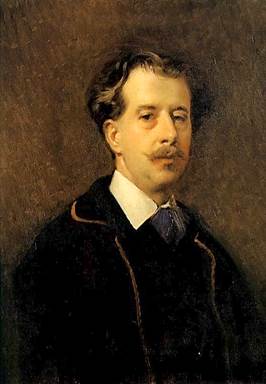This is a detailed portrait painting of a Caucasian man with light skin and a serious facial expression. He has medium-length wavy brown hair and a matching light brown handlebar mustache, accompanied by a small amount of hair beneath his bottom lip. His eyes appear puffy under the lower lids.

He is depicted wearing a black jacket with contrasting trim—gray, gold, or red—suggested by various descriptions. Underneath, he dons a white collared shirt with what seems to be a blue tie, cravat, or vest partially obscured by the jacket. His small lips and slightly rounded, less defined chin also add to his distinctive features.

The man's shoulders are somewhat slumped, and his body is oriented towards the right, captured in a three-quarter profile. This orientation, combined with the light source coming from the left, highlights one side of his face more prominently. The background of the painting features a rich mocha brown color with shades of gray, creating a mottled and slightly smudged effect that blends with the edges of the subject towards the bottom of the image. This nuanced backdrop further emphasizes the central figure without distinct borders.